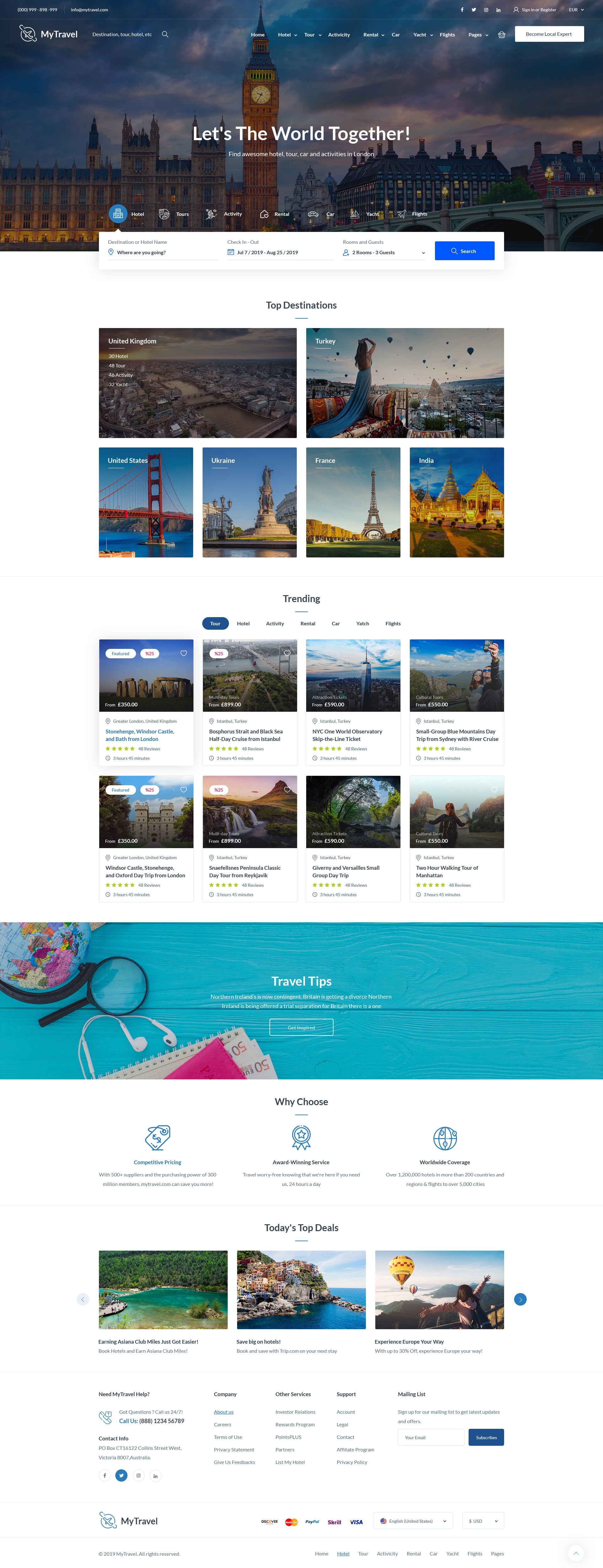The image features a nighttime view of what appears to be a prominent London landmark, possibly Buckingham Palace, silhouetted against a darkening sky with blue and white clouds. In the upper left corner, there's text in white displaying the phone number "000-999-898-999" and the email address "info@mytravel.com." 

Spanning the middle section, social media icons for Facebook, Twitter, Instagram, and LinkedIn are prominently displayed, followed by the options to "Sign In" or "Register." The currency "EUR" is noted alongside a thin white line with a magnifying glass icon, adjacent to the text "My Travel Destination" and options for "Tour," "Hotel," and more.

Across the top, white text lists navigation options: "Home," "Tour," "Active City," "Rental Car," "Yacht," "Flights," and "Pages." A white rectangle contains the call-to-action "Become Local Expert" in black text. Further down, a slogan reads "Let's The World Together, Find Awesome Hotel, Tour, and Activities in London."

A series of images showcases top travel destinations: the United Kingdom, Turkey, the United States (featuring the iconic red San Francisco bridge), Ukraine, France, and India. Below this, categories labeled "Trend" include "Tour," "Hotel," "Activity," "Rental Car," "Yacht," and "Flights."